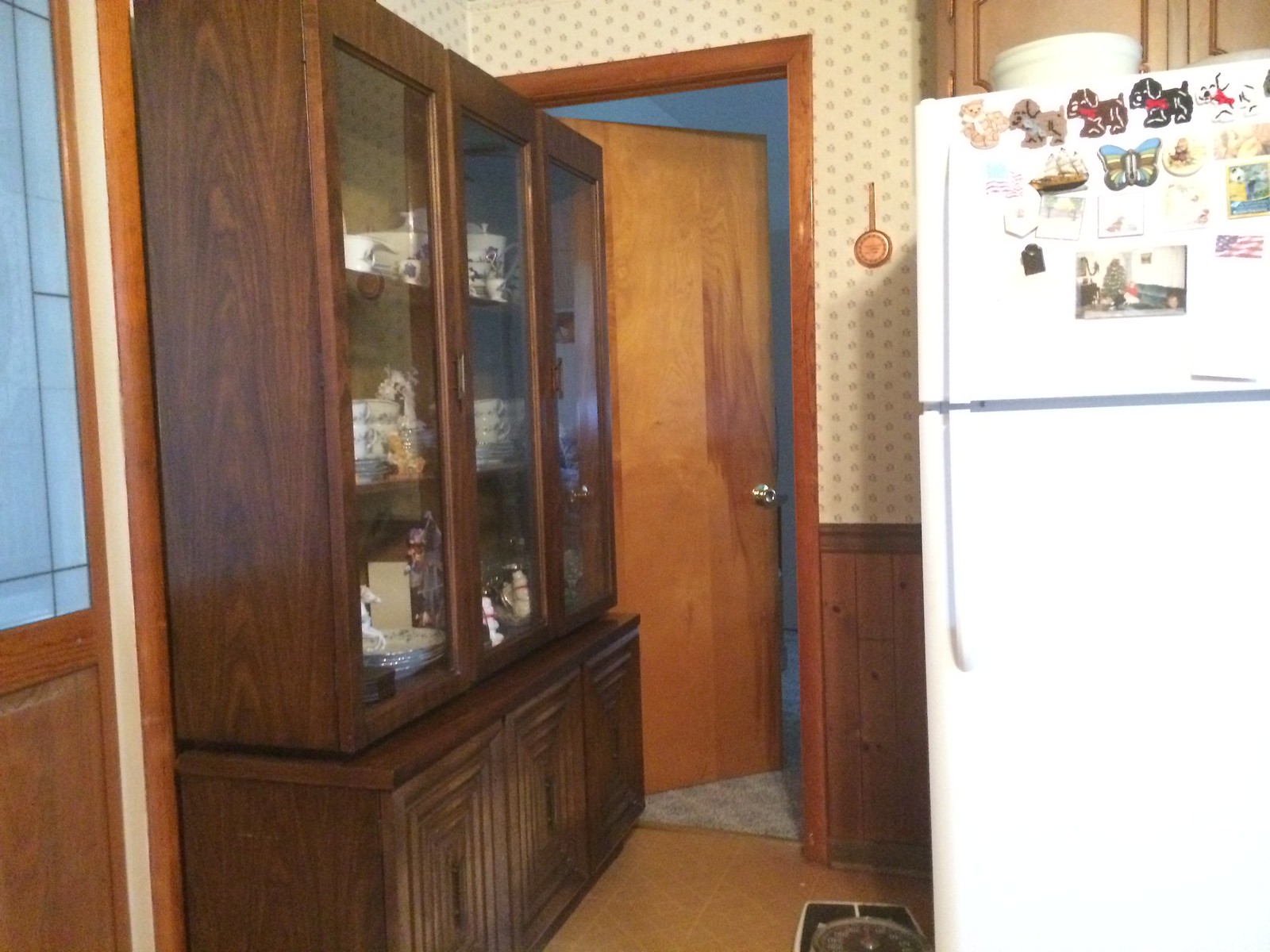The photograph prominently features a corner of a kitchen with a focal point on a large wooden cabinet and a refrigerator. The dark brown wooden cabinet, positioned on the left, has three glass-paneled sections, displaying various ceramic items such as bowls, plates, and cups on two shelves. The bottom part of the cabinet is an opaque section, segmented into three parts, housing additional dining ware. The cabinet stands against a wall that features a dual design; the top half adorned with white wallpaper speckled with black dots and the bottom half lined with brown wooden boards. 

On the right side of the image is a refrigerator adorned with an assortment of magnets and photos. The upper freezer door showcases dog-shaped magnets, a butterfly magnet, a picture of an American flag, and various photos, while the lower refrigerator door remains uncluttered. Above the fridge, a wood cabinet further complements the kitchen's brown-toned theme. In the background, there's a door slightly ajar, suggesting an entryway to another room, and to the left of the main cabinet, another door leads outside. The scene is set against a brown tiled floor, completing the warm, earthy ambiance of the kitchen.